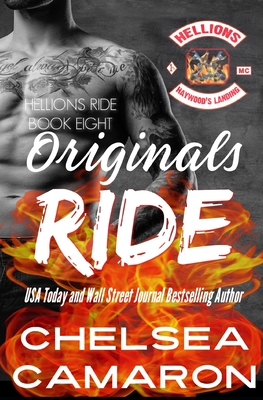The image is a dramatic black and white book cover featuring a muscular, tattooed man from his chin down to his shorts. His chest, neck, and arm are adorned with intricate floral and textual tattoos. The cover prominently displays fiery elements with vibrant yellow, red, and orange hues at the bottom, creating a striking contrast against the monochrome image of the man. Across the center of the man's chest, bold text reads "Hellions Ride, Book 8," with "Originals Ride" written in a large, eye-catching white outlined in red marker font. Below this, the cover highlights the accolades "USA Today and Wall Street Journal Best-Selling Author" and the author's name, "Chelsea Cameron," in white. In the upper right corner, there's a fireman’s emblem with the text "Hellions Haywood Landing" in red, adding a distinctive touch.